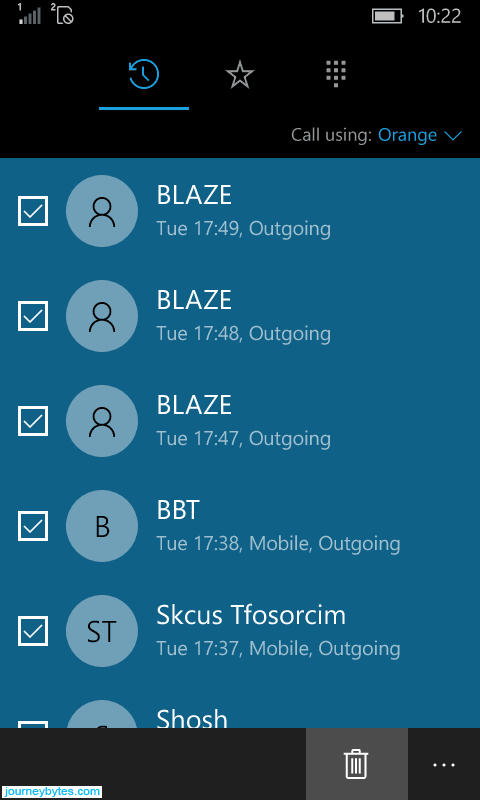This image captures a screenshot from a cell phone, with visible indicator icons along the top edge, including a battery level at approximately 80%, and the time reading 10:22. In the navigation bar, there is a clock with an arrow, indicating an active selection. The central portion of the screen is highlighted in teal, displaying the text "Call using Orange".

On the far left, there are multiple checkboxes, which are all marked. Adjacent to these checkboxes, there are circular icons depicting various elements. Each icon is followed by text and timestamps, detailing outgoing calls.

- The first entry includes a check mark and an avatar icon (a simple head and shoulder outline), with the contact name "Blaze" and details "Tuesday 17:49 outgoing".
- The second entry similarly has a check mark and the same avatar icon, with the same contact "Blaze" and "Tuesday 07:48 outgoing".
- The third entry repeats this format, displaying "Blaze" and "Tuesday 07:47 outgoing".
- The fourth entry, marked with a "B" in the circle, lists "BBT" and "Tuesday 07:38 mobile outgoing".
- The final legible entry shows a check mark, with the name "ST Ciscus Chephoricum" and "Tuesday 17:37 mobile outgoing".

The final entry visible on the screen is partially cut off but includes the text "shoo shoo".